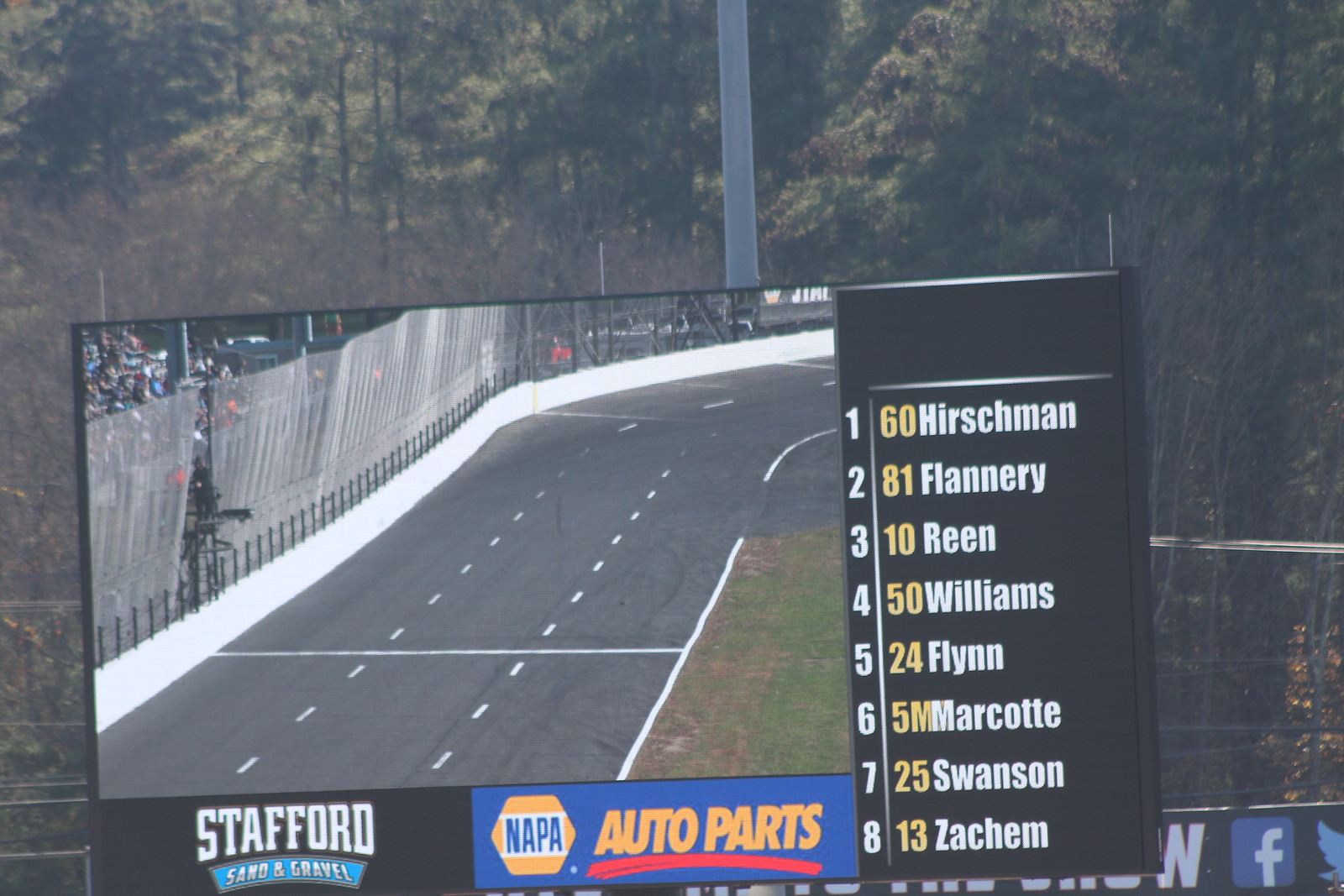This photograph captures an outdoor setting featuring a large video board displaying a racetrack scene. The racetrack, visible on the screen, comprises three lanes separated by white lines, encircling a grassy area, and is bordered by a white barrier topped with black iron and a screening fence that stretches several feet between the track and the audience, some of whom are visible towards the back. Surrounding the board are trees that frame the background.

On the right side of the screen is a list of names ranked from 1 to 8, which are: 60 Hirschman, 81 Flannery, 10 Reen, 50 Williams, 24 Flynn, 5M Marcotte, 25 Swanson, and 13 Zayachim. Below the list, at the bottom of the screen, corporate logos and names are displayed, including advertisements for Stratford Sand & Gravel, rendered in white text on a black background with a blue banner, and for Napa Auto Parts, in yellow, blue, and red. Additionally, a Facebook symbol can be seen in the bottom right corner of the board.